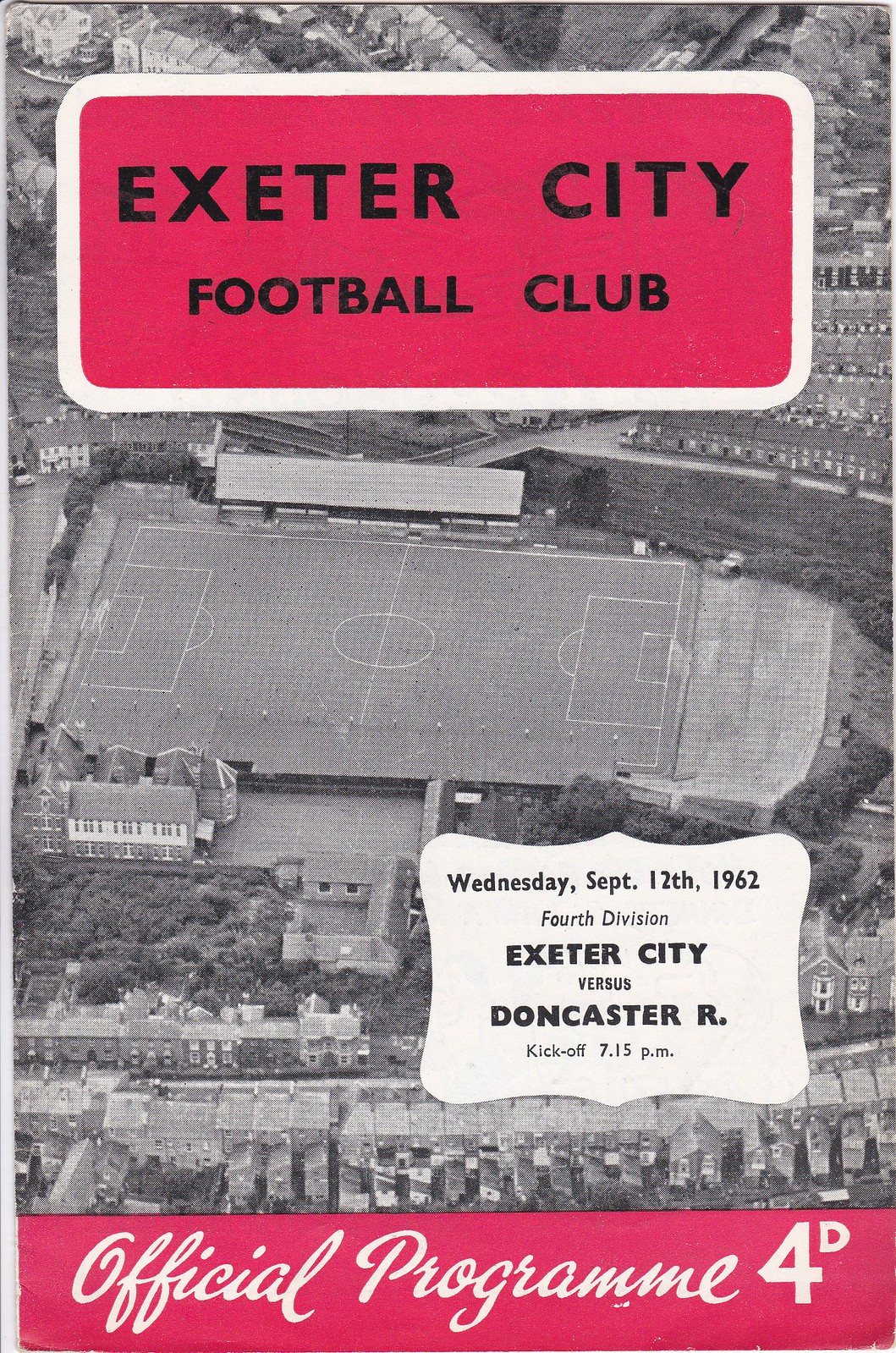The front cover of this European football program features a bird’s-eye view of a soccer stadium and surrounding houses, all rendered in black and white. At the top of the cover, a red text box with a white border displays "Exeter City Football Club" in bold black letters. On the bottom right, a white text box provides match details in black letters: "Wednesday, September 12th, 1962, 4th Division, Exeter City vs. Doncaster R., Kickoff 7.15 p.m." Running along the bottom is a red band with the text "Official Program 4D" in elegant white cursive.